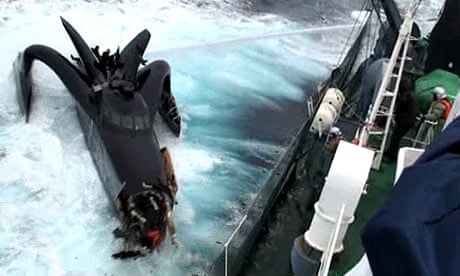In this turbulent scene, we see a partially visible large ship on the right side of the image, possibly involved in a rescue operation, as indicated by its crane and various items aboard. The details offer glimpses of white structures and other equipment aboard the ship. A figure of a man, dressed in a life jacket and wearing a helmet, stands indistinctly in the foreground to the right, adding a sense of urgency to the scene.

On the left side, the focus shifts to a striking black watercraft, drawing comparisons to Batman's motorboat due to its unusual and futuristic design. This boat features a streamlined, elongated shape with the front end severely damaged, broken, and resembling a hydrofoil craft meant for high-speed travel. Its design includes peculiar wings or fins on its sides that curve and bend outward, giving it a serpentine appearance. The central part of the craft has a protruding cabin area with small windows, enhancing its sleek yet mysterious look. The water around the boats is extremely choppy, filled with tumultuous waves and white caps, indicating either natural turbulence or the aftermath of an ongoing event. This compelling combination of details and elements creates a dramatic and vivid portrayal of a chaotic scene on the water.